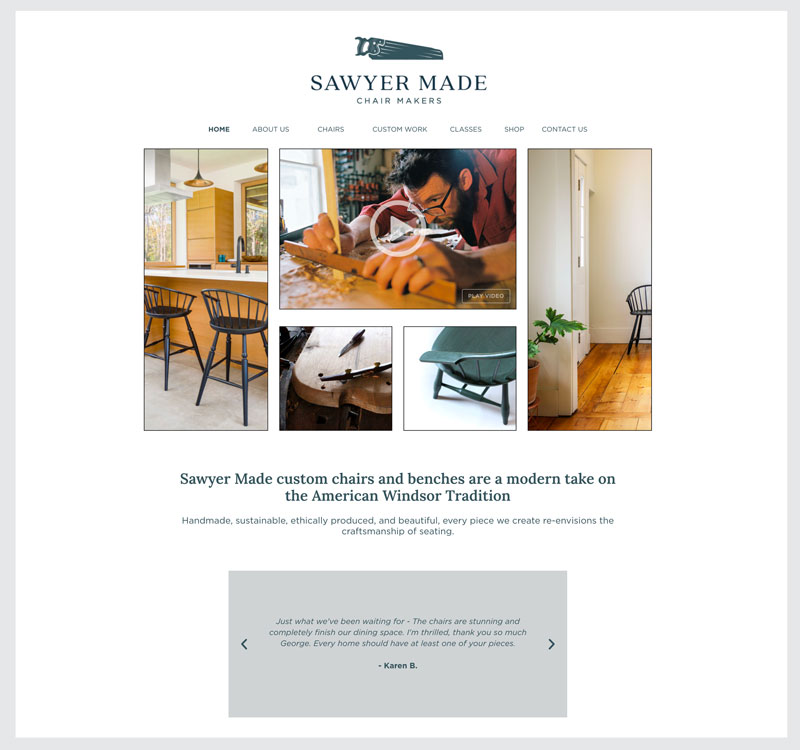The screenshot captures a webpage from "Sawyer Made Chair Makers," identifiable by its logo featuring a hand saw at the top center. Below the logo, the text "Sawyer Made Chair Makers" is prominently displayed in blue. The navigation menu spans horizontally from left to right, including tabs for Home, About Us, Chairs, Custom Work, Classes, Shop, and Contact Us. Centrally aligned beneath these tabs are six images and a video thumbnail. The images predominantly showcase chairs placed on tile floors, likely within kitchen settings, and the video appears to depict a person engaged in woodworking. The webpage's main text states, "Sawyer Made Custom Chairs and Benches are a modern take on the American Windsor Tradition," in blue font on a white background. Below this text, there is a grey box with arrows, which may contain a carousel or additional information. The webpage's overall color scheme includes blue, white, brown, yellow, and green, creating a visually appealing and professional presentation.